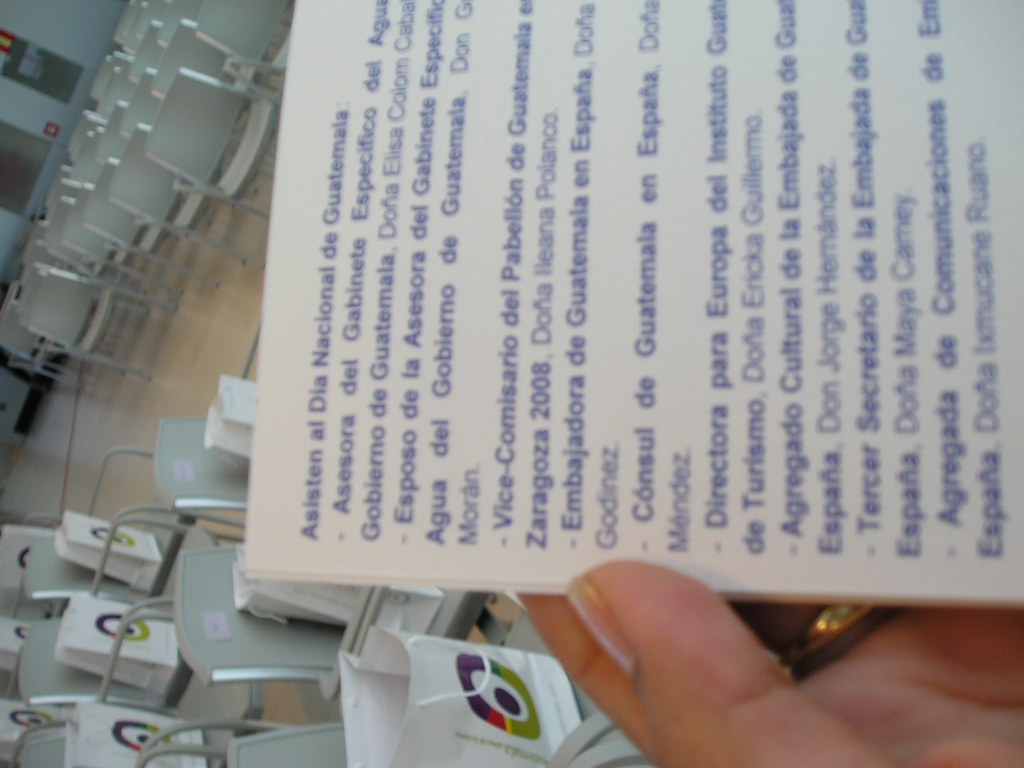The image captures an auditorium with a smooth, shiny wooden floor and whitewashed walls. Rows of gray chairs fill the space, and the chairs on the left side are adorned with colorful gift bags, each marked with an 'O' symbol featuring a purple dot in the center. The 'O' symbols vary in color, including purple, pink, green, yellow, and orange. There's a distinct aisle running through the middle, separating the chairs on the left from the empty chairs on the right. In the foreground, a woman's hand, wearing a golden ring, holds a piece of paper with text in Spanish. The top of the paper reads "ASISTEN AL DÍA NACIONAL DE GUATEMALA." The meticulously arranged setting, highlighted by the organized chairs and neat placement of gift bags, suggests a well-prepared event or gathering.